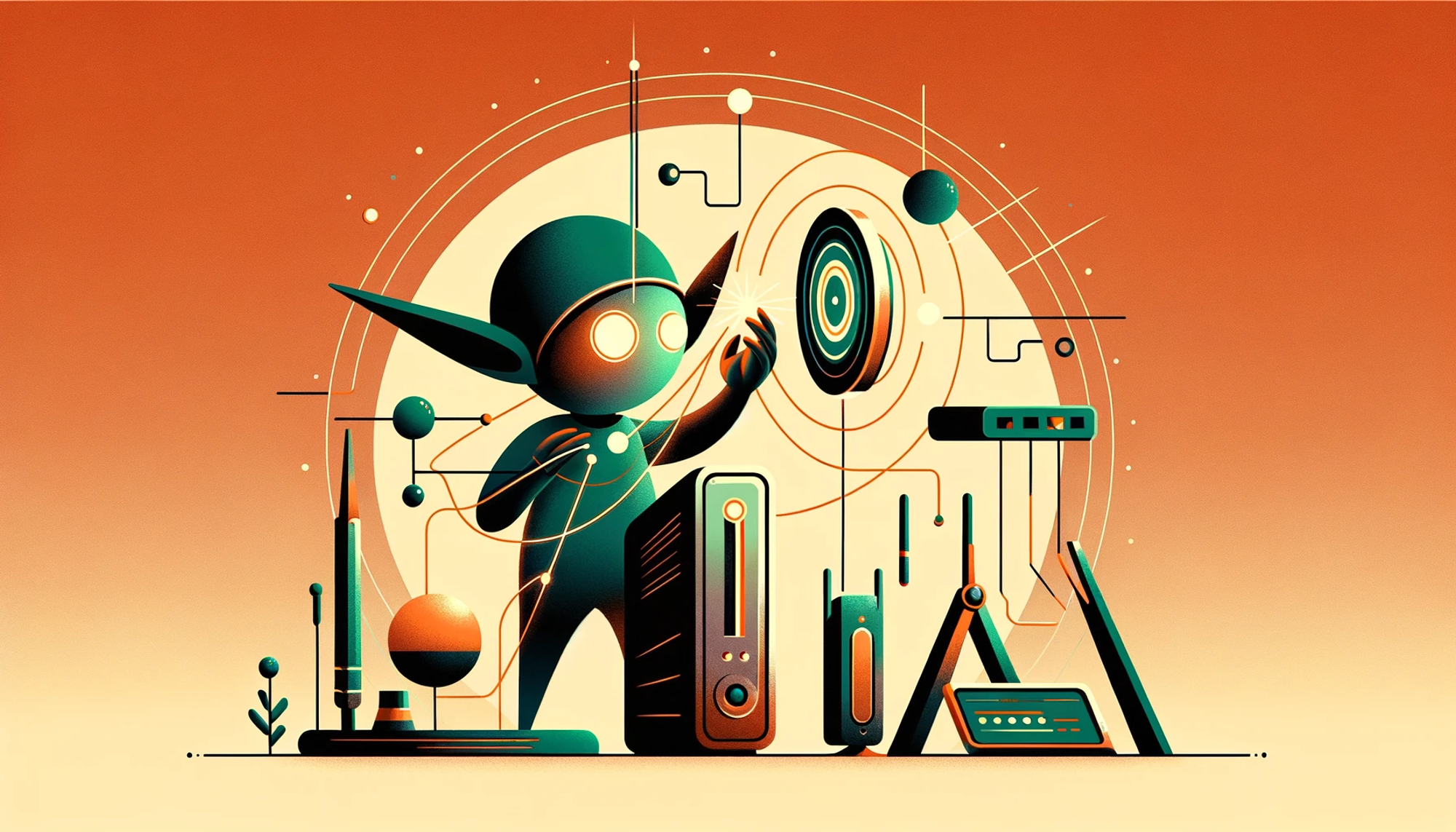The vibrant, possibly AI-generated image showcases a futuristic scene with rich visual details. At the top, a deep orange hue transitions down in ombre layers to a pale creamy yellow at the bottom. Dominating the center is a larger cream-colored circle reminiscent of the moon, surrounded by fine concentric circles and a sprinkling of white dots. Emerging from this central circle are several spikes.

In front of the backdrop stands an alien creature with long, pointy ears, exuding vivid green hues with touches of orange on its helmet, face, and arms. The creature's wide, round, white eyes lend it a striking, otherworldly presence. Adjacent to the alien figure, towards its right, is a dartboard-like object with multiple colored rings including white, green, and orange, centered with a bullseye.

At the feet of the alien rests what appears to be a computer CPU. To its left, a collection of objects likely representing scientific instruments can be seen, among which is an artificial plant-like structure made of green materials. Further to the right, a series of electronic devices are present, including items resembling a router and an iPad, enhancing the futuristic ambiance.

The entire scene is peppered with elements hinting at an alien civilization or a high-tech laboratory, complete with tripods, circuit-like diagrams, and a variety of peculiar scientific apparatuses, merging elements of sci-fi and early 20th-century art styles into a single, intricate tableau.